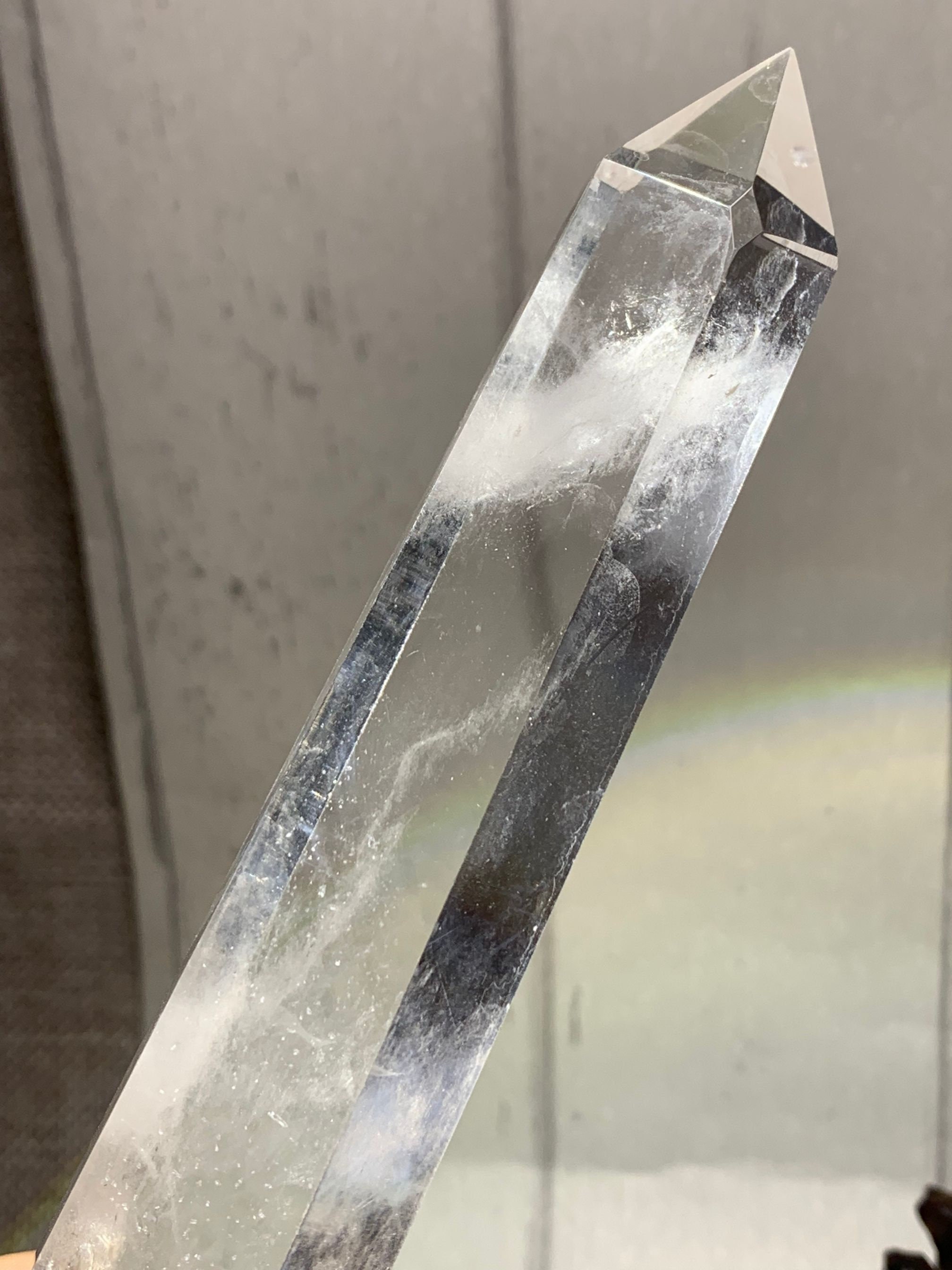The photo showcases a large, clear crystal, prominently positioned diagonally from the bottom left to almost the top right corner, resembling an obelisk with a pointed, pyramid-like tip. The crystal, with its several straight, flat facets, appears transparent but contains cloudy white shatters or lines within. It is set against a background of white, wooden planks, possibly part of a worn building, adding to the rustic ambiance. A small, indistinct black mark is visible in the bottom right corner of the image, while a subtle, colorful rainbow graces the middle right side, adding a touch of whimsy to the otherwise minimalist composition.